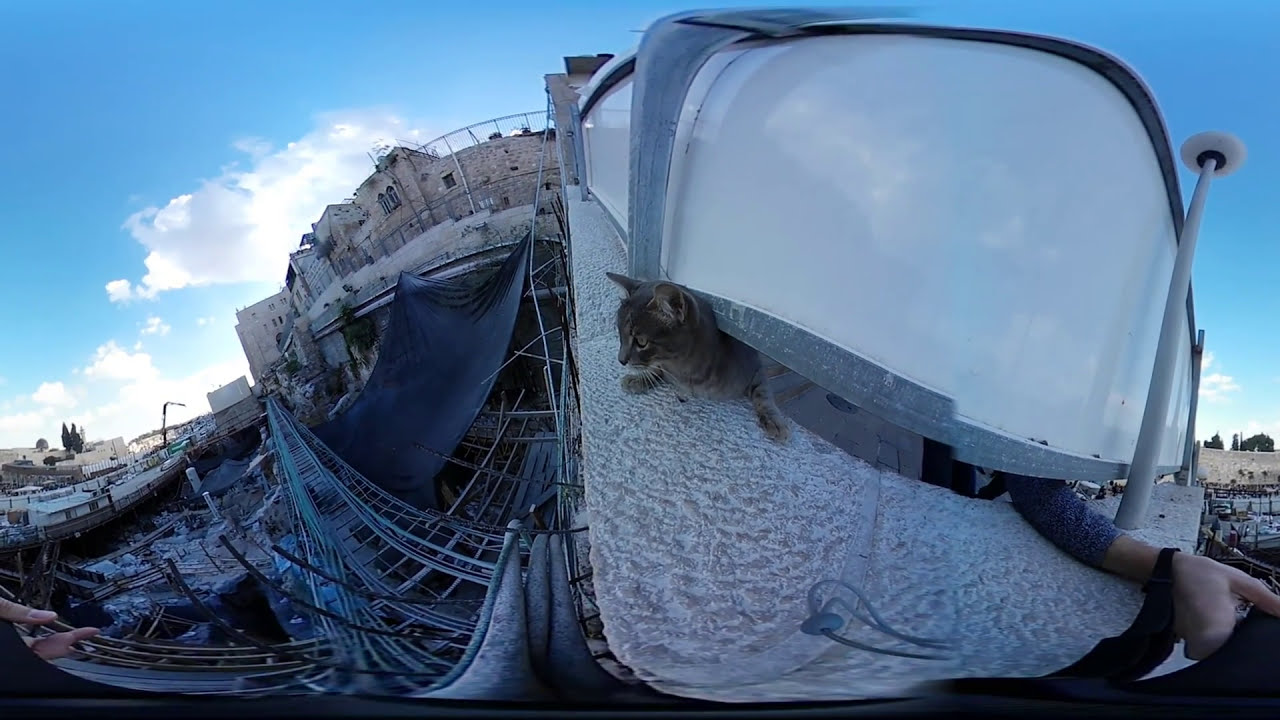The image captures a chaotic outdoor scene centered around the wreckage of an old, dilapidated building. In the foreground, there's a cat perched on a surface, partially covered by a large tarp or protective covering, which also drapes over what appears to be a man's arm reaching out from underneath. The cat is prominently placed in the center of the image. Surrounding this central focus are the remains of a building that appears to have collapsed, with sections of old cement, windows, and what looks like broken wiring scattered about. The sky above is a deep blue with some scattered clouds, suggesting a clear, sunny day. The overall impression is one of disarray, with the collapsed structure and the mixed objects creating a strikingly congested visual.